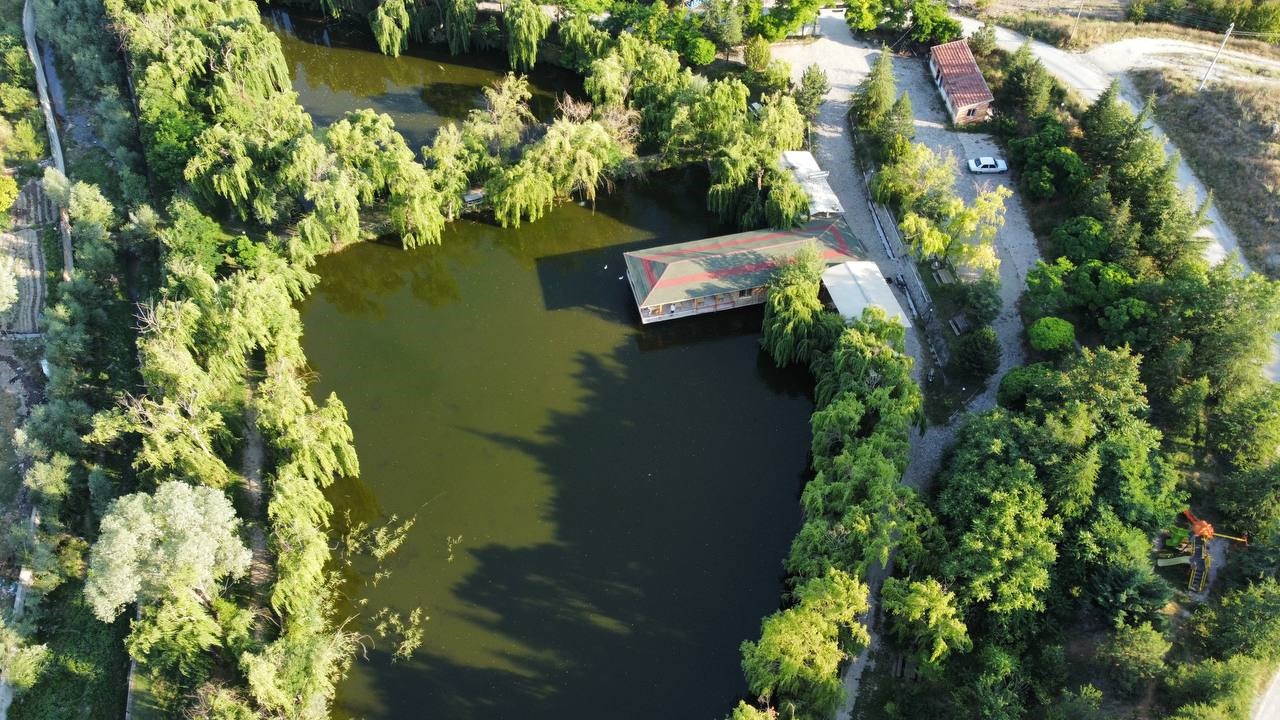This aerial image captures a verdant landscape featuring a central green, mossy pond of irregular shape, surrounded by dense groves of tall trees and varied shrubbery. The scene is bathed in sunlight, enhancing the forest olive green hue that dominates the area. To the right of the pond, a building with a tan roof, accented by a red box structure, juts into the water. Flanking this building are two others with white roofs extending horizontally left and right. A road wraps around these structures, characterized by a central median lined with large trees. This road forms a turnaround area, diverging into additional pathways. In the upper right corner, there is a parking area with a white car. Further out, more roads and grassy meadow areas are visible, devoid of human presence, underlining the serene, natural setting.